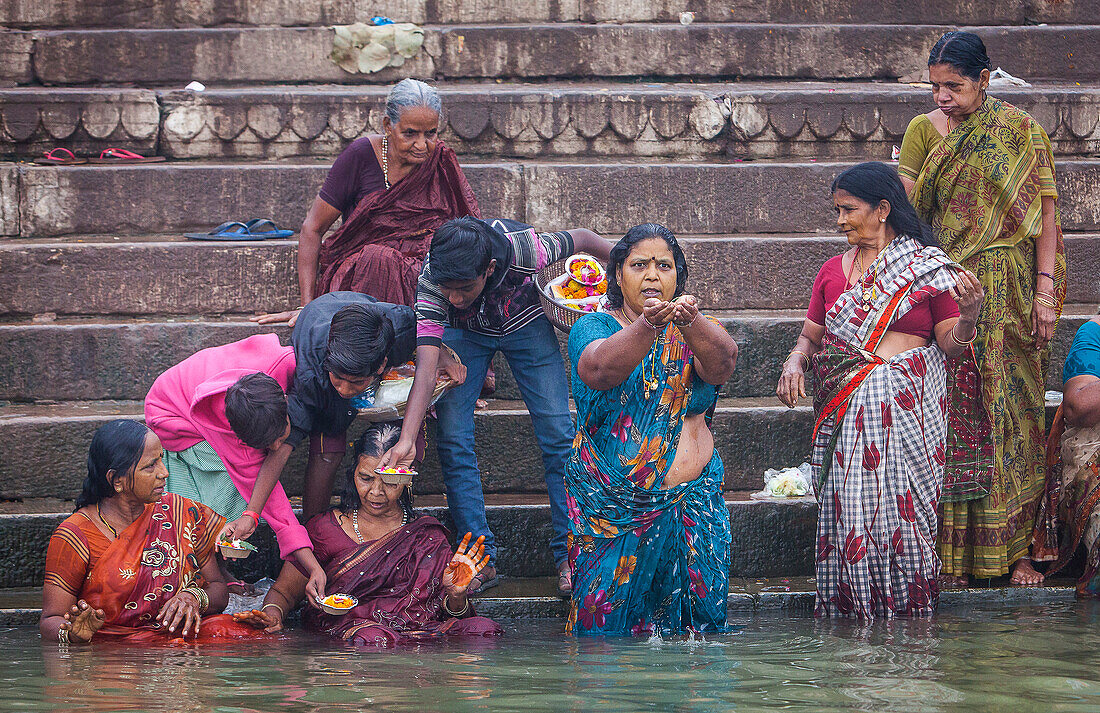In this vibrant image, several women, fully adorned in brightly colored, decorative clothing, are bathing in a body of water surrounded by stone or concrete steps that extend from the water's edge at the bottom all the way to the top of the scene. On the left side, two women are seated in the water, wearing exceptionally bright attire, as young boys lean towards them, offering flower petals from small trays. A boy in jeans holds a basket, possibly containing fruit, just behind these women. Behind them, an older woman sits on the steps. Towards the center and right of the image, three more women can be seen, two standing in the water, and one on the lowest step just before entering the water. There's an additional glimpse of a person seated further to the right. Of special note, one of the seated women to the left is displaying her palm, which is dyed darkly, potentially with henna. The scene is a tapestry of color, movement, and cultural activity set against the backdrop of the earthy, brownish-gray steps.